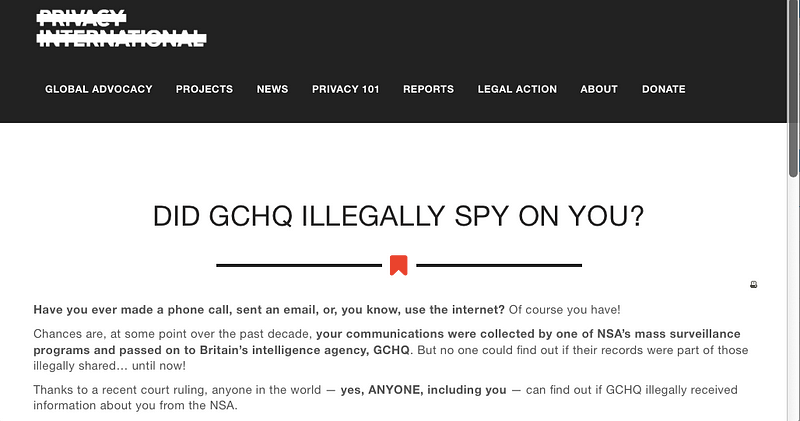The image shows a webpage from Privacy International with a black banner at the top featuring white text. The banner includes sections titled Global Advocacy, Project News, Privacy 101, Reports, Legal Action, About, and Donate. Below the banner, the main content is presented on a white background with black text that highlights recent developments concerning the surveillance activities of the UK's Government Communications Headquarters (GCHQ).

The headline reads, "Did GCHQ illegally spy on you?" followed by a series of questions: "Have you ever made a phone call, sent an email, or used the internet?" The text explains that over the past decade, the NSA's mass surveillance programs likely collected your communications and could have shared the data with GCHQ unlawfully. A recent court ruling now makes it possible for anyone, anywhere in the world, to determine if GCHQ received their information from the NSA.

The document provides more details as you scroll, but the initial section emphasizes the significance of the court's decision and its potential implications. The web design itself is minimalistic, primarily utilizing black text on a white background, with a notable detail: the phrase "Privacy International" is visually struck through, as if marked with correction fluid. This stark design choice underscores the gravity and controversial nature of the subject matter.